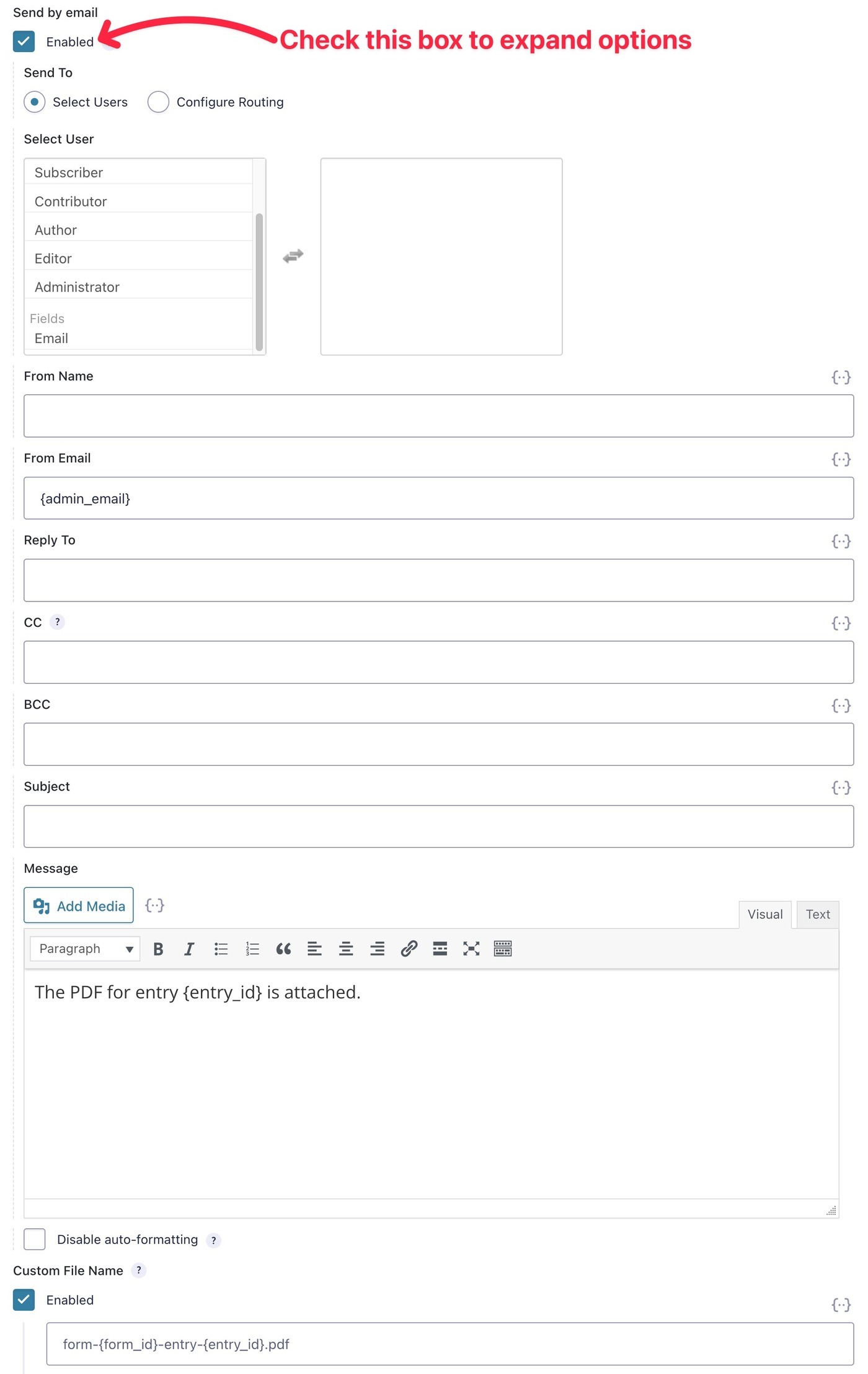Screenshot Description: Messaging App Configuration Interface

The provided screenshot displays a section of a messaging app constructed with a white background. Starting in the upper left-hand corner, bold text reads "Send by Mail." Directly beneath this, there is a square blue icon containing a checkmark, indicating an enabled status. Adjacent to this icon on the right, the term "Enabled" is clearly written.

Centrally located on the page, a dynamic red text message states, "Check this box to expand options," accompanied by an arched arrow that curves leftward, pointing toward the "Enabled" section.

On the left-hand side of the screenshot, two primary options are presented: "Send to Select Users" and "Configure Routing." The "Select Users" option is currently selected, as highlighted. Directly beneath this, there is a designated box where various user types are listed, including "Subscriber," "Contributor," "Author," "Editor," "Administrator," and "Fields," followed by an email address entry.

Beneath the "Select User" section, there are six long, horizontal rectangular input fields stacked vertically. These fields are specified for different email components: "From Name," "From Email," "Reply To," "CC," "BCC," and "Subject."

At the bottom of the page, there is a segment for composing a message, labeled "Message." Within this area, there is an option to "Add Media." The message composition box contains the default text: "The PDF for Entry is attached." Furthermore, there is a section available for specifying a custom file name.